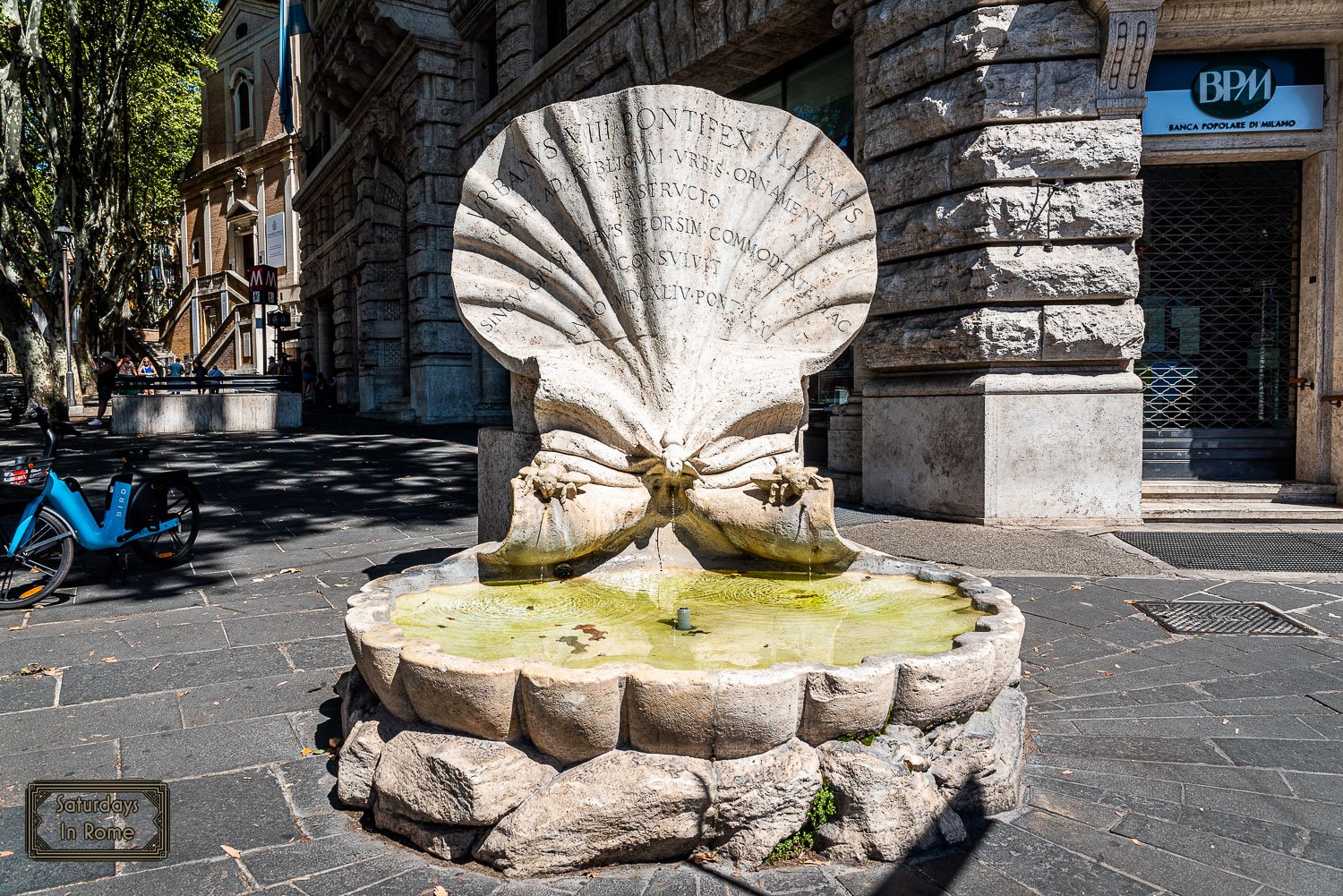The image captures a detailed scene of an ancient fountain located in a downtown area, prominently centered in the frame. The fountain itself features a ceramic or brick base with a shallow, scalloped-edged basin containing water that has a greenish tint, likely due to algae. Rising from the center of the fountain is a large, clam-like structure with text engraved on its curved surface, although the shadows and curvature make the text difficult to read.

Surrounding the fountain is a dark gray brick or concrete surface. To the right, the façade of a stone building is visible, bearing a sign that reads "BPM" above a door, with "Banca Polar de Milano" indicated below, suggesting the scene might be in Italy, specifically Rome, as another inscription in the corner claims.

In the background, there are additional buildings, some with stone finishes, and mature trees, contributing to a clean and structured urban environment. On the left side of the image, a blue e-bike is parked. A manhole cover or grate is also noticeable in the paving. Though not immediately apparent, some people can be discerned in the distant background, adding a touch of life to the otherwise serene historical setting.